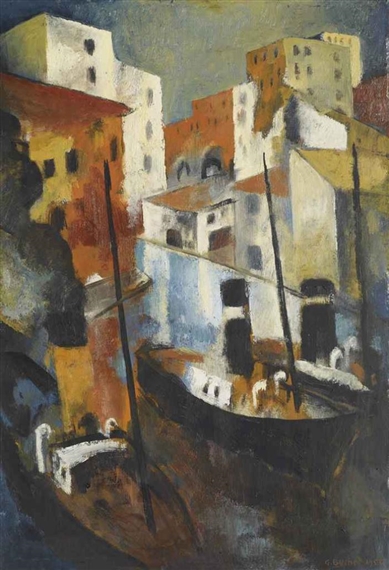The painting depicts a serene waterfront scene, likely reminiscent of Venice, featuring a row of up to three boats set against a backdrop of tall, stucco buildings in varying shades of white and terracotta. The buildings, characterized by their simple, rectangular shapes, partially emerge from the water, enhancing the impression that they stand amidst canals. The boats, resembling gondolas or steamboats, are lined up from the bottom left corner, ascending diagonally to the right. One boat emits smoke from its smokestack, while the others are inactive. The boats exhibit functional elements like pillars for sails but lack actual sails. The water's dark hue contrasts with the buildings and the sky, which sports a blend of light greens, blues, and darker shades towards the edges, with tinges of yellow suggesting a twilight or night setting. This visually rich scene captures the timeless, tranquil essence of a historic, possibly Mediterranean locale.